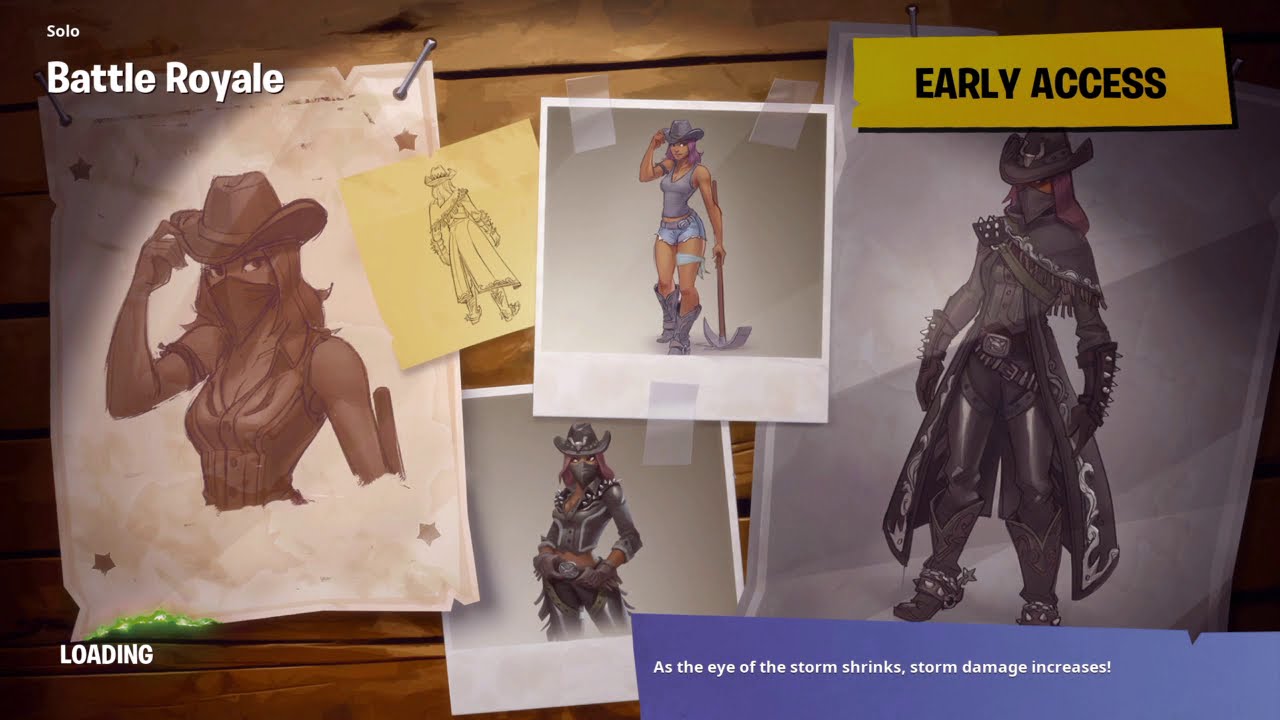The image appears to be a loading screen from a Battle Royale video game. The background is composed of slats of a wood wall. In the upper left corner, white text reads "Solo Battle Royale," and in the upper right corner, black capitalized letters on a yellow rectangular background proclaim "Early Access." Scattered across the screen are various depictions of a female cowboy character, each in a different pose or style. 

On the left side, tacked to the wall, is a detailed sketch of the woman wearing a cowboy hat, a handkerchief covering her mouth, and a tight-fitting tank top, with one hand touching the brim of her hat. To the right of this sketch is a yellow post-it note featuring a black pencil drawing of the woman from behind, showing her long jacket and hat. Further right, there is a Polaroid-style photo taped to the board where the woman, again wearing her hat, is depicted holding a pickaxe in her right hand, dressed in shorts and a tank top, with her left hand touching the brim of her hat.

Minimal text placed on the bottom left reads "Loading" in white capitalized letters. The characters and sketches exhibit a cartoonish style, prominently featuring shades of white, brown, gray, yellow, blue, orange, and green. The bottom right-hand corner carries a white text message stating, "As the eye of the storm shrinks, storm damage increases!" The overall composition and elements suggest this is a screenshot possibly taken from a computer or console, giving the impression of a game's visual thematic design.